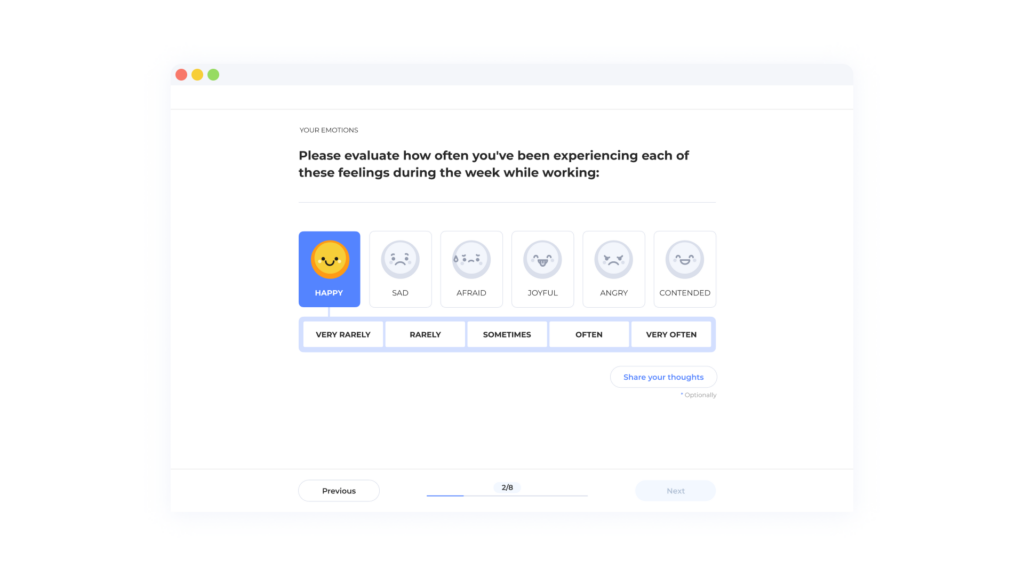The screenshot depicts page two of an eight-page questionnaire from a mobile application designed to assess the emotions individuals experience during their working week. The interface has a clean, white background with a straightforward layout. At the top, bold black text reads, “Your Emotions,” followed by an instruction to “please evaluate how often you’ve been experiencing each of these feelings during the week while working.”

Beneath the instruction, six yellow smiley-face icons are displayed, each representing a different emotion: happy, sad, afraid, joyful, angry, and contented. Each smiley face varies in expression to match the specified emotion. The “happy” emotion has been highlighted with a blue background, signaling it has been selected, while the other five icons remain in a sepia-toned, grayed-out state, indicating they have not yet been chosen.

Below the emotional icons, a selection bar allows users to rate the frequency of their feelings on a scale ranging from “very rarely” to “very often.” 

At the bottom of the screen, there are navigational buttons labeled “Previous” and “Next,” which enable users to move through the eight pages of the questionnaire. Additionally, a button labeled “Share Your Thoughts” is present, presumably allowing users to provide further comments or insights about their emotional experiences.

Overall, the screenshot showcases an intuitive and user-friendly design aimed at capturing detailed feedback on workplace emotions.